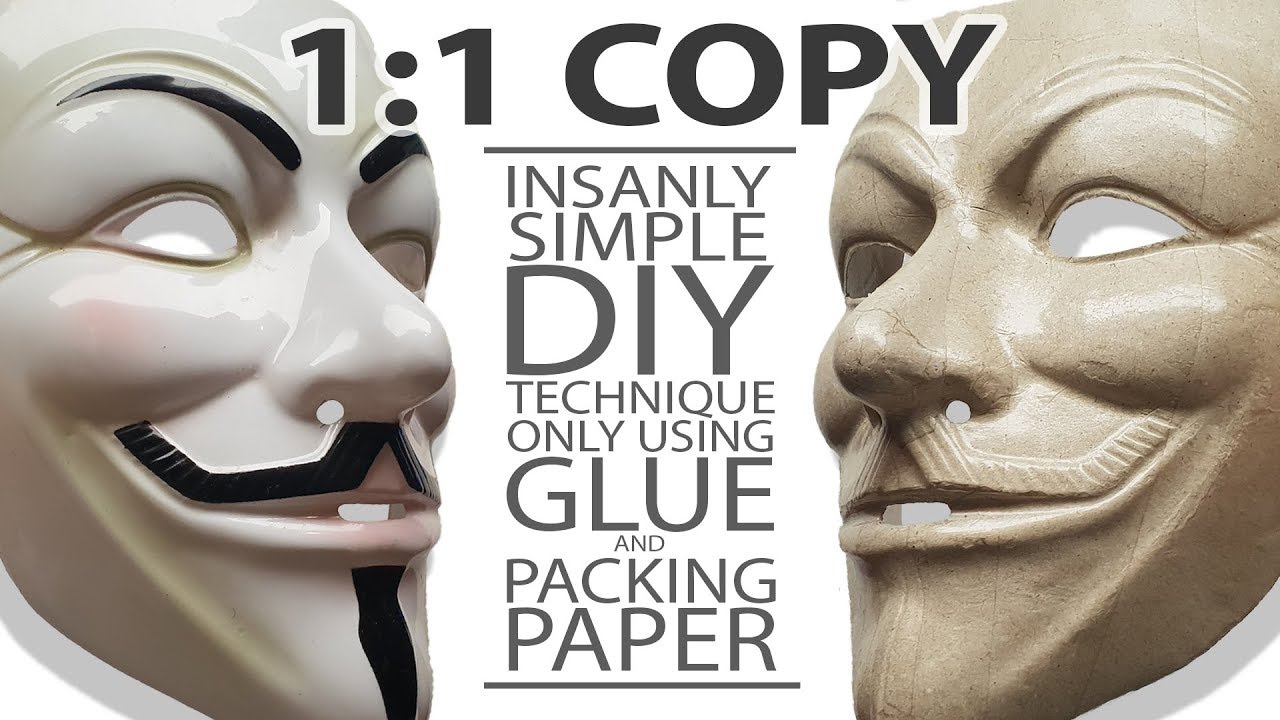The poster features a plain white background with two Guy Fawkes masks prominently displayed on either side. The mask on the left is the traditional version, made of a shiny white ceramic material, with a black mustache, goatee, and eyebrows, pink blush on the cheeks, and eye holes. The mask on the right appears to be an unpainted replica, with a light tan, cement-like texture, retaining the mustache and goatee outlines but without any color. Across the top, in black text, it reads "1:1 copy," followed by a small line. Below this, in a brown font, it states, "Insanely simple DIY technique using only glue and packing paper," with another small line beneath it.